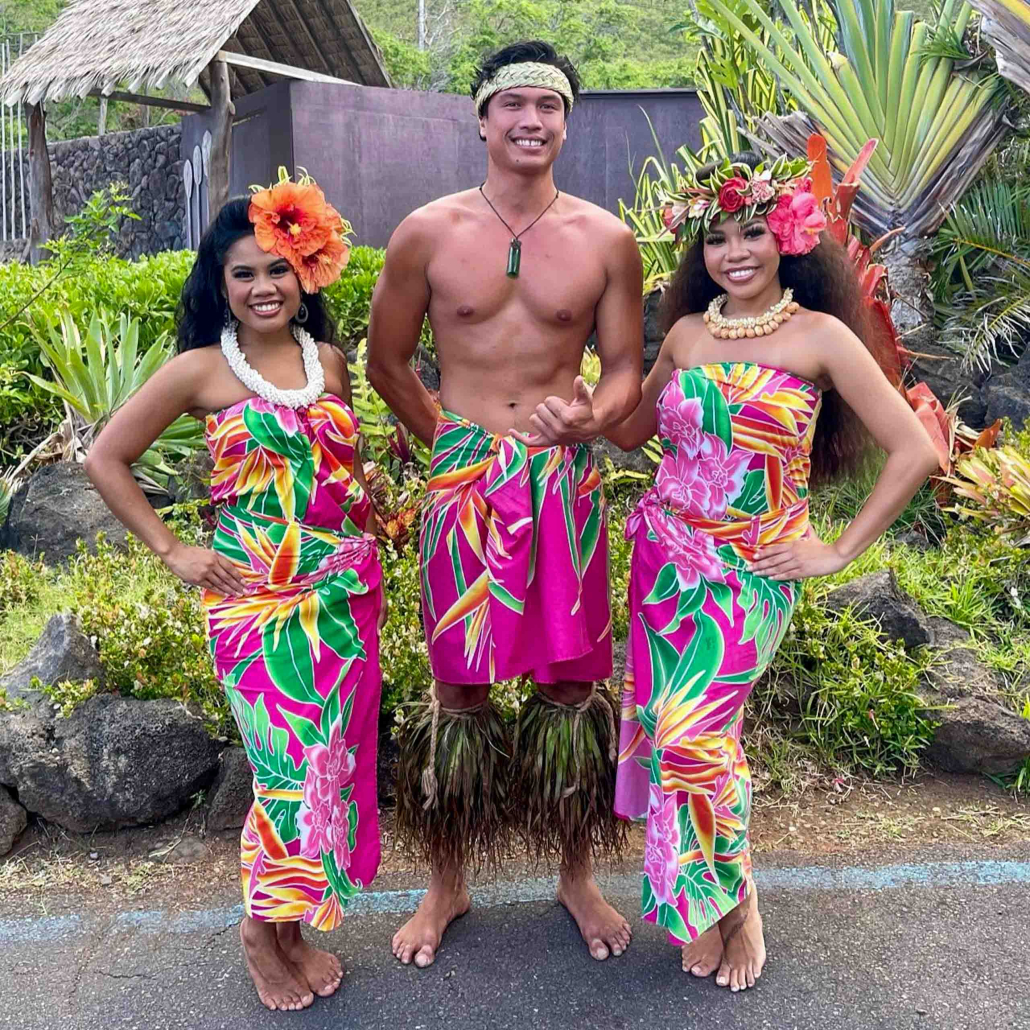In a vibrant tropical setting, three smiling individuals are captured in a lively group photo, possibly taken in a Pacific Island location such as Hawaii, Thailand, or another Polynesian island. Central in the photo is a shirtless man adorned with a woven bandana, a fabric wrap around his waist, and distinctive tropical garb on his shins. Flanking him are two women wearing elaborate floral garlands on their heads and adorned with matching bright tropical dresses featuring a vivid mix of pink, green, yellow, and red patterns, decorated with striking orange flowers. The women have long hair and floral jewelry around their necks, complementing their festive attire. The trio stands in a symmetrical pose with their elbows out, suggesting they're about to perform a traditional dance. The background reveals a tropical garden with lush greenery and palm-like trees, alongside a rustic shed with a rush-built roof, adding to the exotic ambiance of the scene.